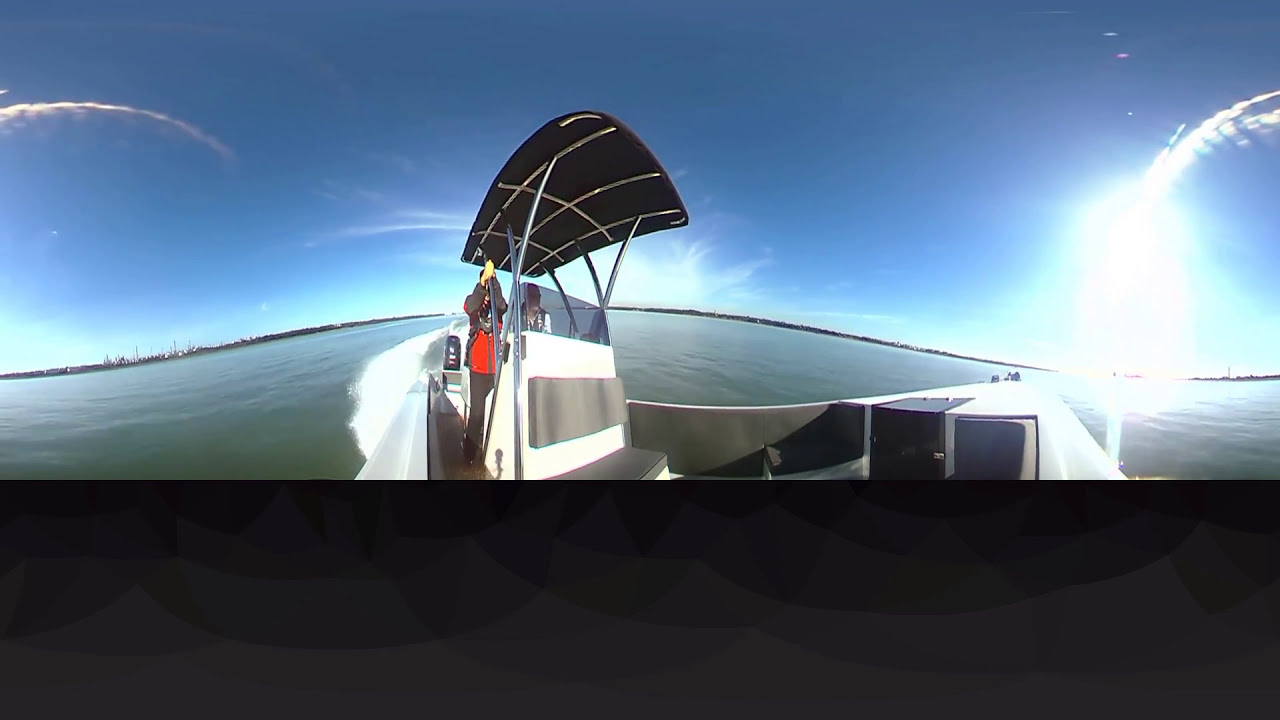The image portrays a boat navigating a large body of water, with two people visible at the console, one of whom is wearing a bright red jacket. The boat, which is white with black accents, has a shaded canopy above the console, providing protection from the sun. The clear blue sky and distant landmass, which includes small structures, suggest a summer setting. The water beneath the vessel is depicted in a dark, murky gray-green color, transitioning to lighter shades near the horizon. A beam of light stretches laterally across the image, enhancing the wavy, warped effect caused by the camera lens. The lower third of the picture is distinctly blotted out in black, obscuring some details of the boat's lower structure. The overall scene encapsulates the movement and activity of the boat on an expansive, possibly oceanic, water body, with bright and dark contrasts emphasizing the vividness and motion.